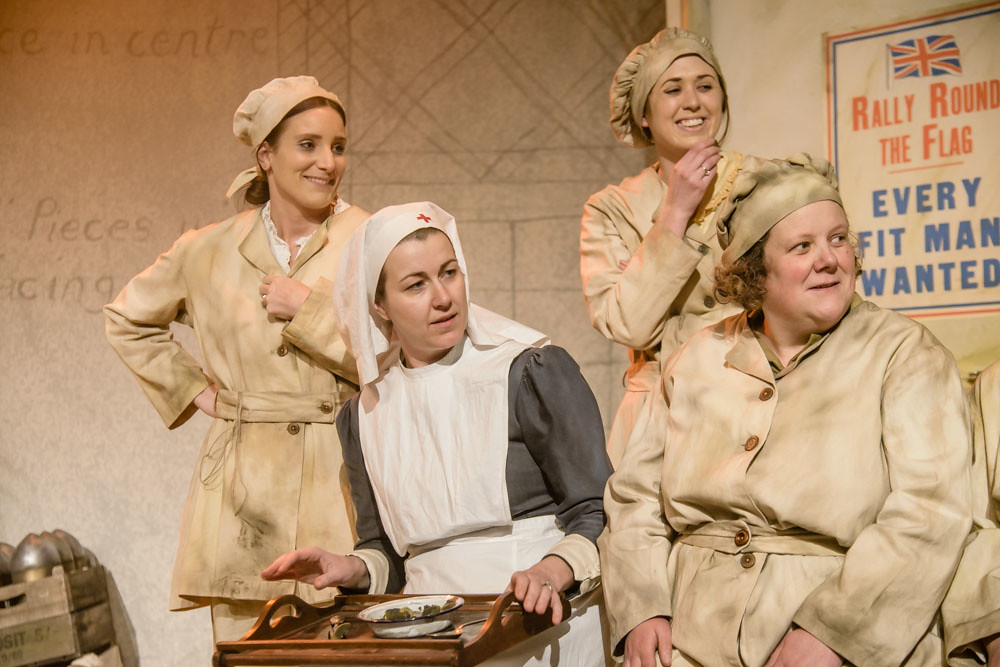The photograph depicts four Caucasian women, likely from England, dressed in historical military uniforms reminiscent of World War II. Three women are clad in tan coats and matching tan hats, while the fourth woman is in a nurse's uniform composed of a gray and white outfit with a hat bearing a Red Cross emblem. She balances a wooden tray laden with food on her lap. All four women are gazing to their left with expressions of amusement. In the background, a box of ammunition shells and a canvas wall adorned with an advertisement can be seen. The advertisement, set against a British flag, reads, "Rally Round the Flag, Every Fit Man Wanted." The overall scene suggests a wartime setting or a re-enactment, capturing a moment that appears both historical and evocative of the camaraderie and responsibilities of women during the World War II era.